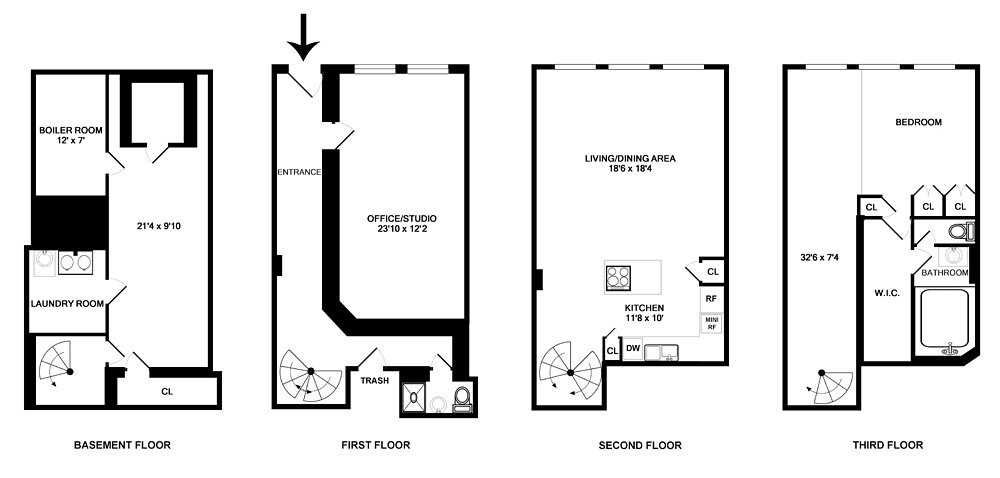The image depicts detailed floor plans for a four-story building, including a basement. Each floor is represented by a separate plan with corresponding labels: basement floor, first floor, second floor, and third floor.

The basement floor plan reveals multiple labeled rooms. In the top left corner, there is a boiler room connected to an unmarked room with specified dimensions. Additionally, the basement includes a laundry room, a small closet, and a space in the bottom left designed for a spiral staircase.

The first-floor plan highlights the continuation of the spiral staircase on the left side, which links all floors. Adjacent to the staircase, you'll find a designated area for trash disposal and a bathroom. A narrow entrance hallway provides access to the main entrance of the building, which in turn leads into a spacious office studio. Essentially, the hallway branches left into the large office and straight ahead to the staircase and bathroom.

On the second floor, the floor plan showcases an expansive open-concept living area with a kitchen. No walls are present, but designated counter space is clearly marked.

The third-floor plan features a somewhat larger hallway that leads to a modestly sized bedroom. This bedroom includes multiple closets and a walk-in closet connected to an adjoining bathroom equipped with both a toilet and a bathtub.